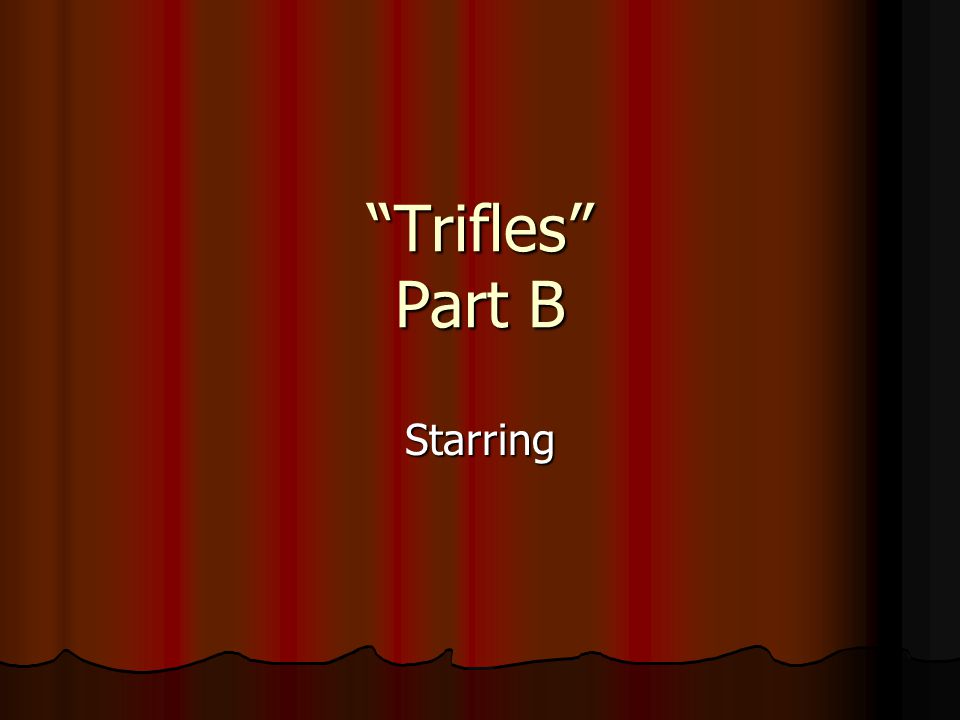The image portrays a stylized stage curtain, predominantly red with highlighted folds in shades of brown and burgundy. The curtain, hanging upright, serves as the backdrop for text which appears centered and horizontal within the composition. At the top of the curtain, in bold beige lettering and enclosed in quotation marks, is the word "Trifles." Beneath it, also in beige, is the phrase "Part B." Below these, the word "Starring," rendered in white, completes the text. The entire graphic, which is a square, evokes the feel of an introduction to a play with its theatrical elements and formal presentation.